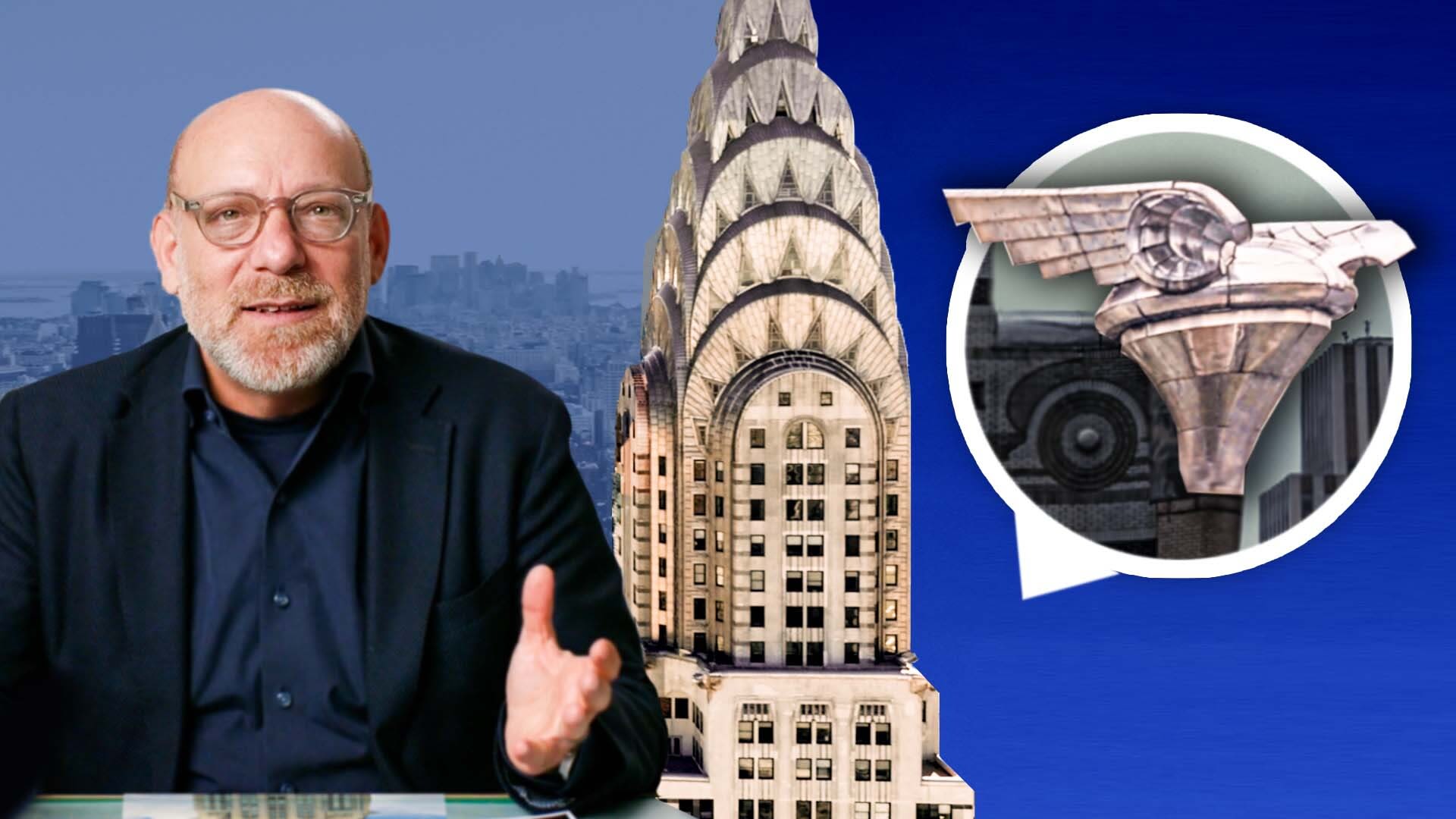The image captures a bald man with glasses, a mustache, and a beard, seated at a glass desk on the left-hand side. He's dressed in a dark-colored jacket over a collared shirt and a t-shirt underneath. He is gesturing with his left hand towards the camera. Behind him is a faded blue cityscape, and in the center of the frame next to him is the top portion of the Chrysler Building from New York City. On the far right, against a flat blue background, there's a white-circled architectural feature with a little triangle at the bottom left-hand side. This highlighted element resembles a classical corbel and is part of the building's intricate design, possibly evoking imagery reminiscent of winged shoes from mythology. This scene, possibly a still from a video or TV show, gives the impression that the man might be explaining or discussing architectural elements.